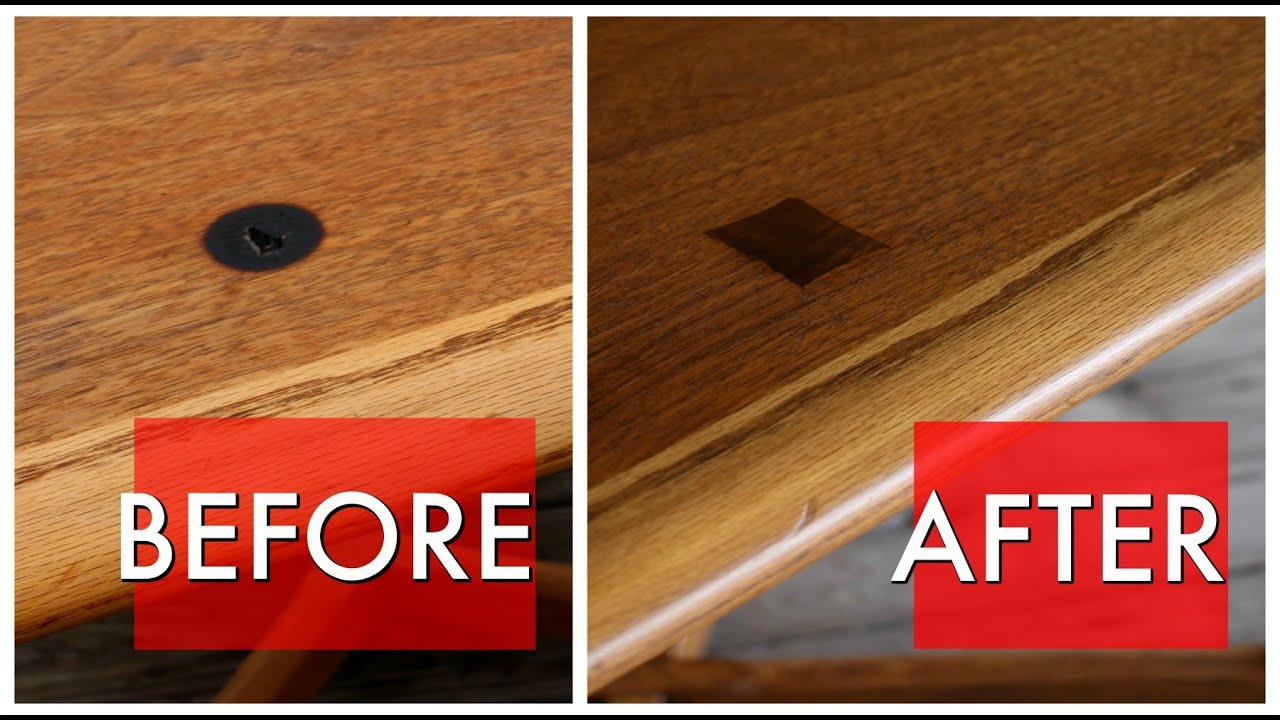This image features a side-by-side comparison of a wooden table labeled "Before" and "After." On the left side, the "Before" photo, marked by white text within a red square, displays a medium-colored wooden table with a conspicuous circular burn mark, which includes a hole at its center. The table surface appears dull and damaged. On the right side, the "After" photo, also labeled with white text in a red square, showcases the same table after repair. The previously burnt and damaged section has been replaced with a darker square patch that seamlessly covers the original hole. The repaired table surface looks shinier and cleaner, highlighting the quality of the restoration work. No other objects or colors are present in the image, focusing attention solely on the table and the repair process.